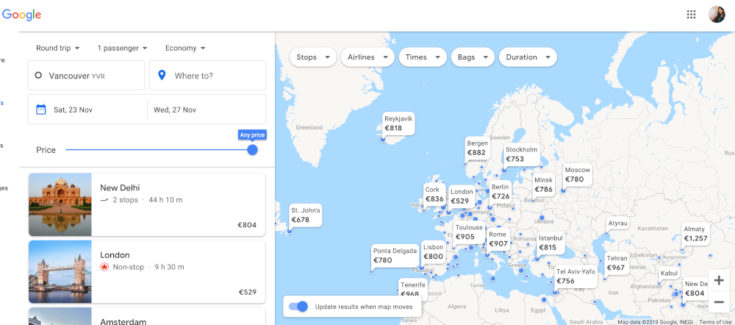The image showcases the interface of a Google search for booking flights. The layout is a horizontal rectangle and features multiple elements to aid users in finding flights.

In the top left corner, the iconic word "Google" is displayed in Google's signature colors: green, blue, red, and yellow. Below this, gray text indicates the search criteria: "round trip, one passenger, economy."

Further down, two adjacent boxes prompt user input: the first box, with a white background, contains the departure city "Vancouver," while the second box is labeled "Where to." 

Underneath these input boxes, a calendar icon is followed by the text "Saturday, 23 November to Wednesday, 27 November," specifying the travel dates. Next to the dates, in small gray text, is the word "Price," which is accompanied by a bright blue banner. This banner, ending with a circle, indicates the filter "Any Price" in white text inside the blue bubble.

Below these filters is a vertical list displaying travel options: New Delhi, London, and Amsterdam. Each city is likely accompanied by travel details such as prices.

On the right side of the image, a world map is populated with small white text bubbles indicating various location names and prices. Situated at the bottom of the map is a toggle button labeled "Update Results when map moves," which is currently turned on.

This detailed interface allows users to input their travel preferences and view a variety of destination options and prices in a visually organized manner.